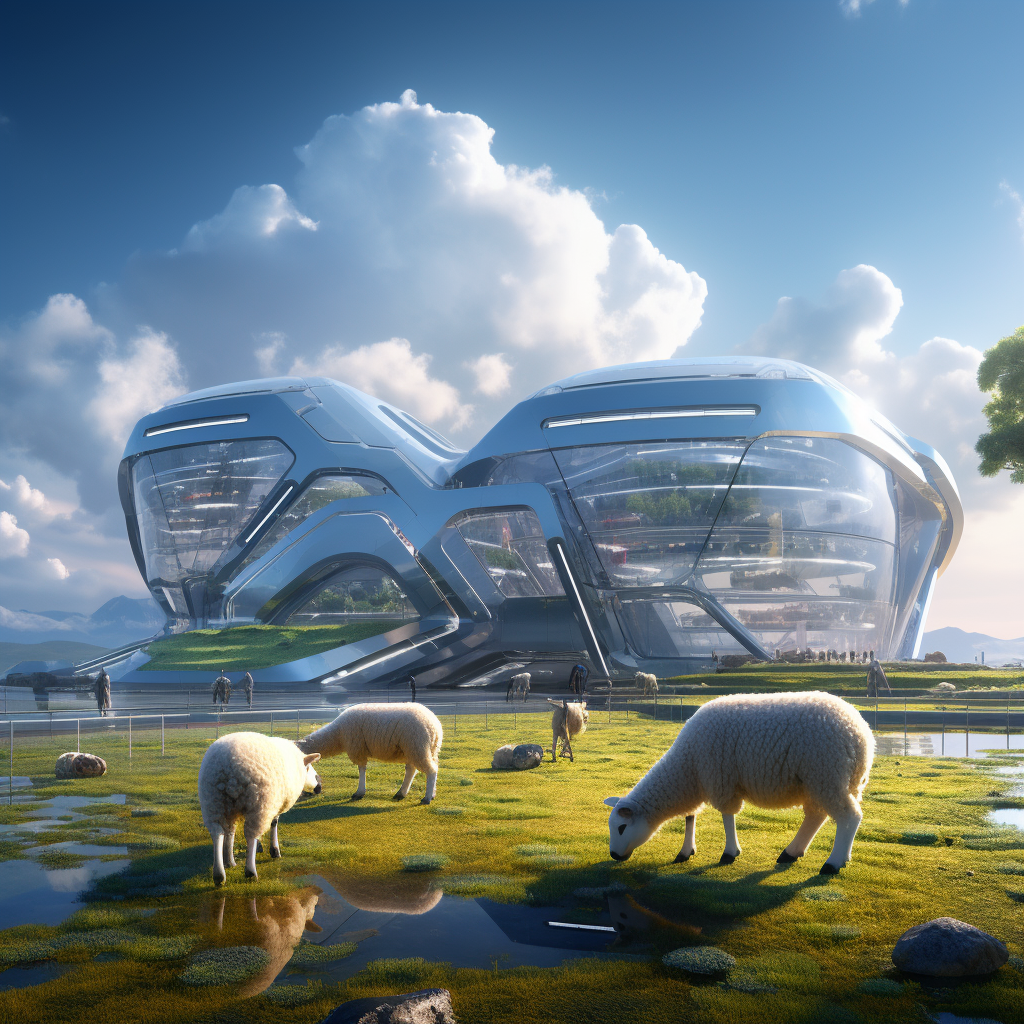In this digitally-rendered image of a futuristic farm, a strikingly bright blue sky adorned with big, puffy white clouds provides a vivid backdrop. Prominent in the background are mountain ranges that lend a natural contrast to the ultramodern architecture in the scene. Dominating the midground is a curvaceous, metallic building with a primarily blue facade and extensive glass windows. Standing approximately four to five stories high, this structure features multiple levels and looks like a blend of a greenhouse and a vast warehouse, hinting at its capacity to house various activities or animals.

In the immediate foreground, a green, wet grassy field dotted with puddles following a recent rain hosts about five to six sheep grazing contentedly. Surrounding the grazing area is a fence that keeps the sheep enclosed. The field also shows signs of other animals, possibly horses or llamas, in the distance. Towards the front, people navigate through paved pathways around the sheep, adding a bustling, communal element to the tranquil pastoral setting. The overall combination of technology and nature portrays an intriguing, nearly otherworldly farm scene.